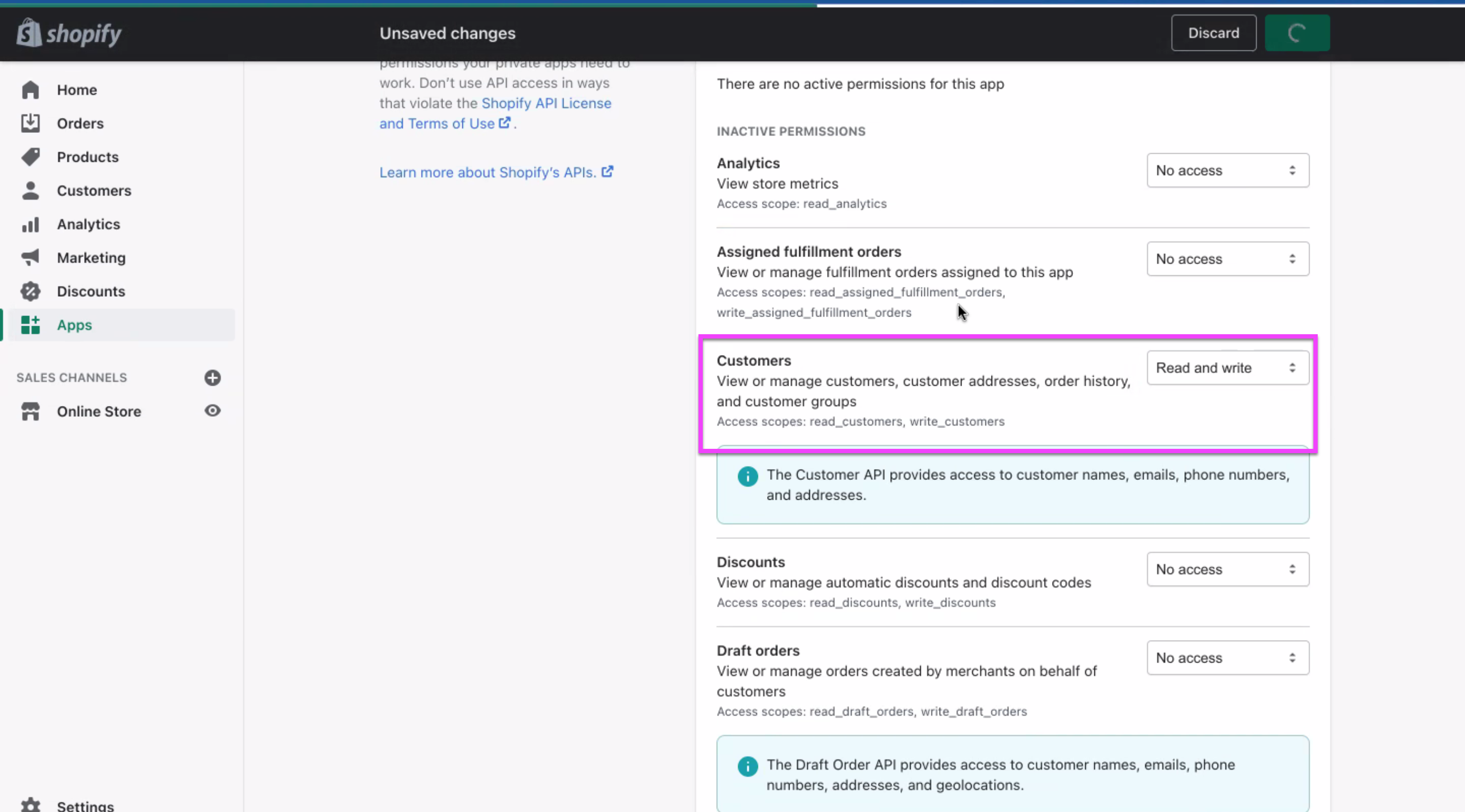**Detailed Caption:**

This image is a screenshot from the settings section of a Shopify storefront. The top banner is black and prominently features the Shopify logo, consisting of a green shopping bag with a white "S" on it, next to the word "Shopify." To the right of the logo, there's a notification stating "unsafe changes," and further to the right is a "Discard" button. Beside it is a green button with a loading circle indicating some ongoing process.

On the left-hand column, beneath the Shopify logo, there are menu options including Home, Orders, Products, Customers, Analytics, Marketing, Discounts, and Apps. Below these, there's a Sales Channel section featuring the "Online Store" option.

Centrally, the main content is displayed against a white background, showcasing the settings under the "Apps" section. It indicates that there are no active permissions for the currently selected app. Inactive permissions are detailed, divided into categories such as:

- **Analytics**: View store metrics, marked as "No Access."
- **Assign Fulfillment Orders**: This includes viewing or managing fulfillment orders assigned to the app, also labeled as "No Access."
- **Customers**: Involves viewing or managing customers, their addresses, order history, and customer groups, which are granted "Read and Write" access.

This section is highlighted by a purple rectangle, drawing attention to the permissions setup.

Beneath this, the "Customer API" is described, granting access to customer names, emails, phone numbers, and addresses. Another section outlines permissions for "Discounts," which includes managing automatic discounts and discount codes, set to "No Access."

Further down, permissions for "Draft Orders" are detailed, including viewing or managing orders created by merchants for customers, again noted as "No Access." It also mentions that the draft order API provides access to customer names, emails, phone numbers, addresses, and geolocations.